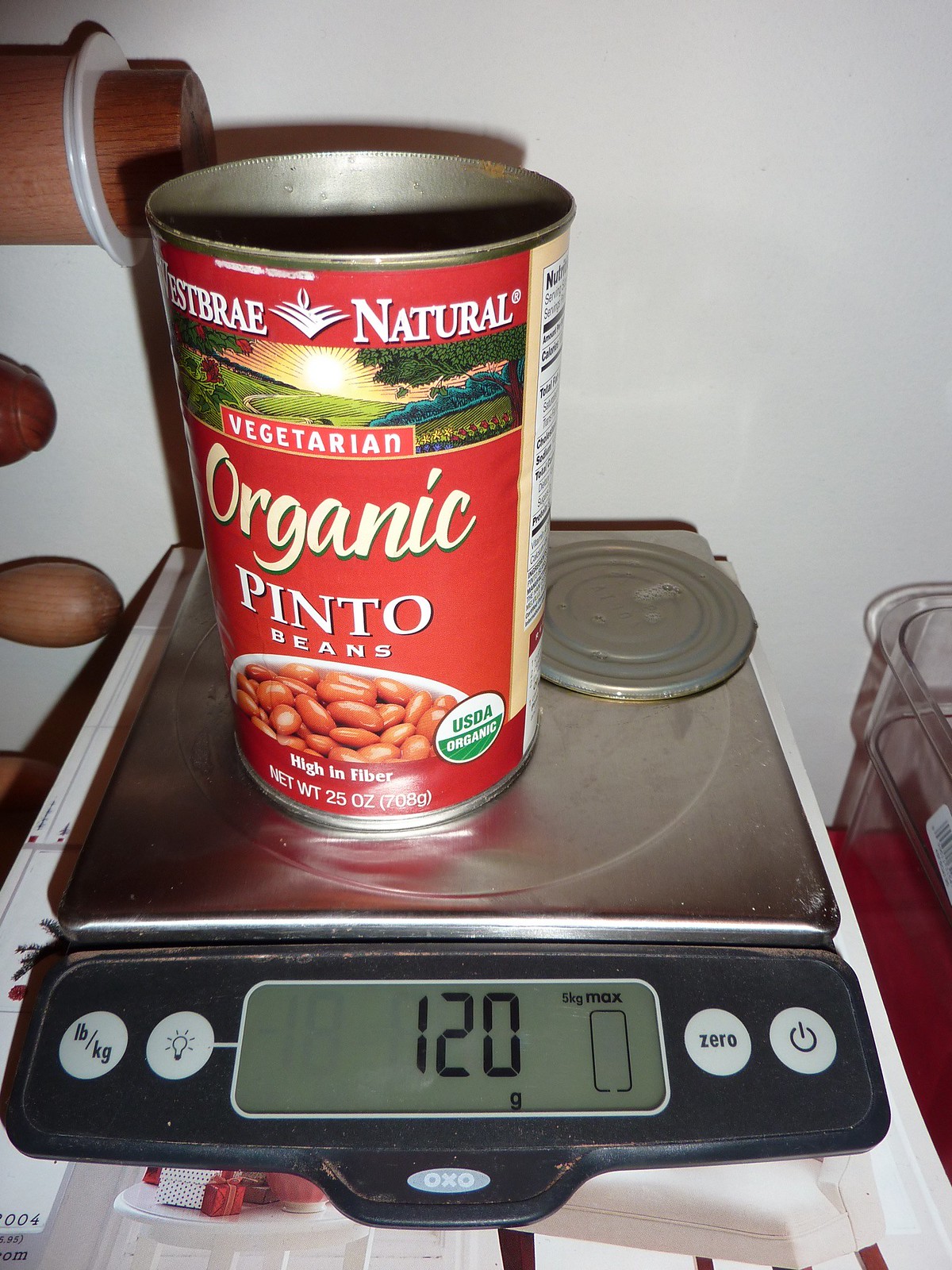This close-up photograph features a 25-ounce can of West Bray Natural Organic Vegetarian Pinto Beans placed on a metal food scale. The can has been opened with a can opener, and the detached metal lid rests on the scale alongside the can. The scale displays a reading of 120 grams. To the right of the scale, there is a clear plastic container, which is empty. The background of the image is a white wall, providing a clean and neutral backdrop that highlights the primary elements in the foreground.